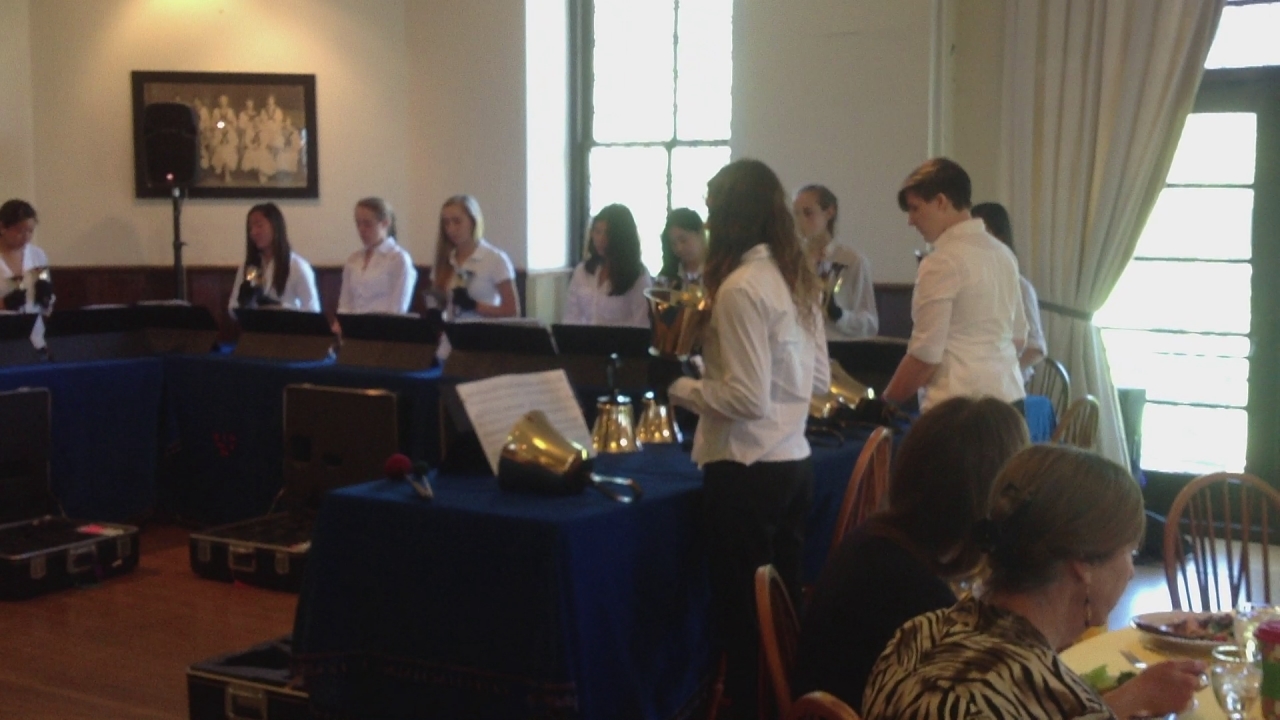In this indoor image set around midday, a central scene unfolds on a hardwood floor. At the heart of the picture is a group of individuals, predominantly dressed in white shirts, standing behind rectangular tables adorned with blue tablecloths. They appear to be part of a musical ensemble, as they are handling large, gold bells or chimes. Flanking the center, there are people seated at a round table in the lower-right corner with plates, cups, and glasses of water, suggesting a mealtime setting. The backdrop reveals large windows draped with heavy curtains, contributing to the overall ambiance. Additional elements include a framed photograph hanging on the wall and open briefcases positioned near the musical tables. The image captures a colorful palette featuring hues of white, off-white, yellow, gray, black, blue, brown, green, and gold, thereby enriching the visual narrative.